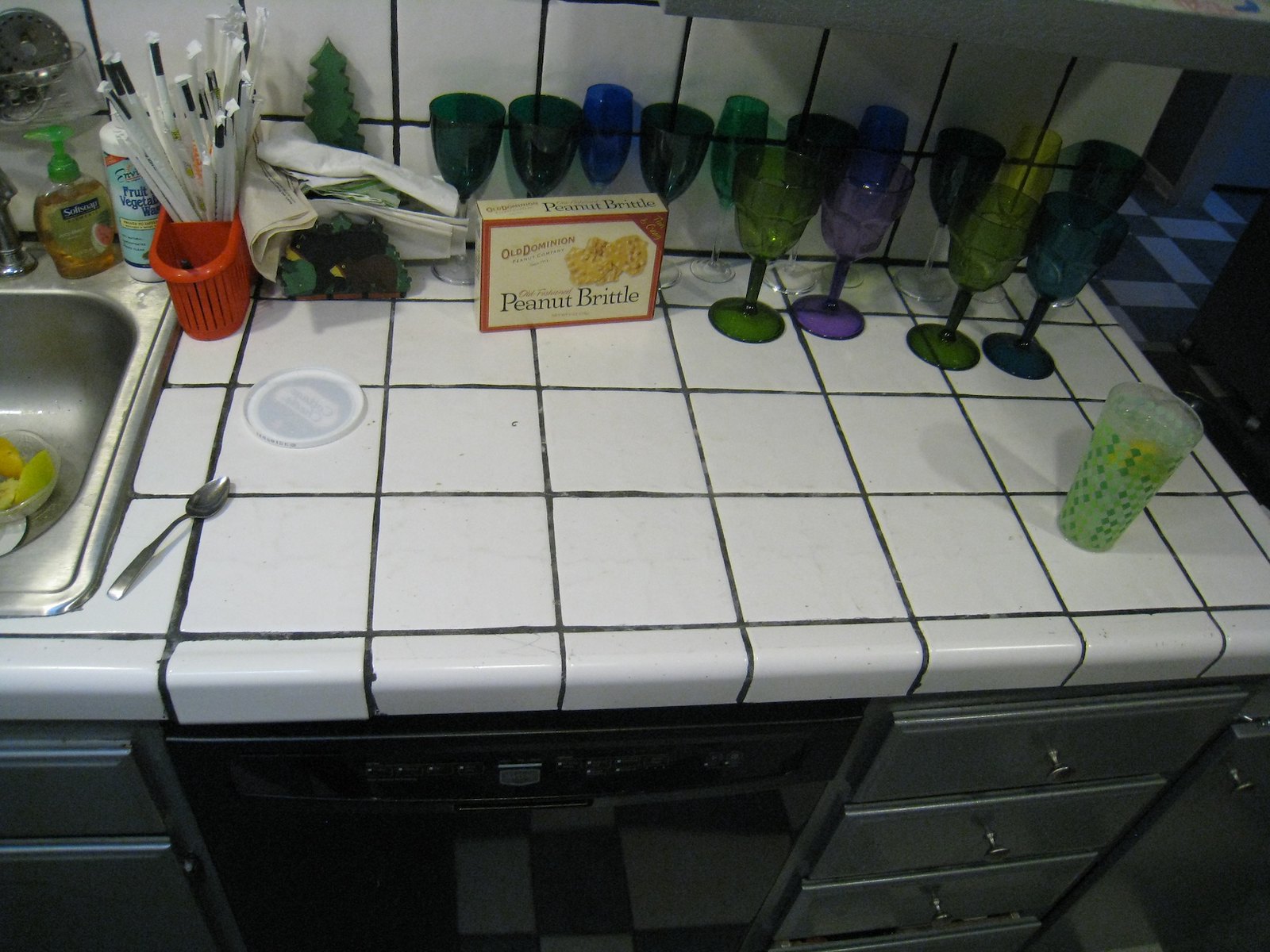This overhead photograph captures the intricate details of a meticulously arranged kitchen counter. The counter itself is composed of white tiles grouted with dark gray, creating a sharp, clean contrast. On the left edge of the photo, a stainless steel sink is partially visible, adorned with a container of soft soap marked by its distinctive green top.

To the far right of the countertop, at the very corner, stands a drinking glass. The glass features a unique diamond-shaped pattern in shades of green, adding a touch of elegance to the scene. 

Lined up against the white-tiled backsplash, a dazzling array of wine glasses catches the eye. These glasses boast deep, rich jewel tones—emerald green, sapphire blue, amethyst purple, and ruby red—each one gleaming with brilliance.

In front of this vibrant display sits a rectangular box of Old Dominion peanut brittle. The box is beige, bordered in red, and showcases an inviting image of two pieces of peanut brittle on its right side.

Finally, a lone spoon lies diagonally, with its handle resting beside the sink and pointing towards the right side of the photograph, completing this visually engaging kitchen tableau.